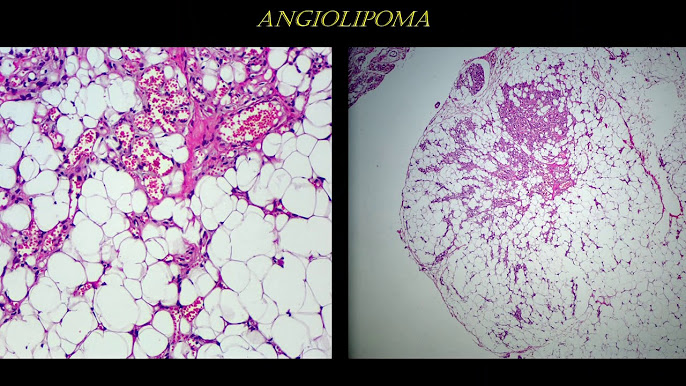This image features two side-by-side microscopic photographs set against a black background. At the very top, in italicized yellow uppercase text, the label "ANGIOLIPOMA" is prominently displayed. Both images, illustrative of angiolipoma, share a similar composition of pink, white, and purple elements. The left image presents a highly magnified view, showcasing a complex network of white areas interspersed with pink and purple lines and dots, resembling cells and veins. The right image, though similar in content, offers a more zoomed-out perspective, revealing larger sections of the same intricate pattern, with more pronounced open white spaces. This detailed visual study highlights the cellular structure and distribution, possibly indicating characteristics of a medical condition.